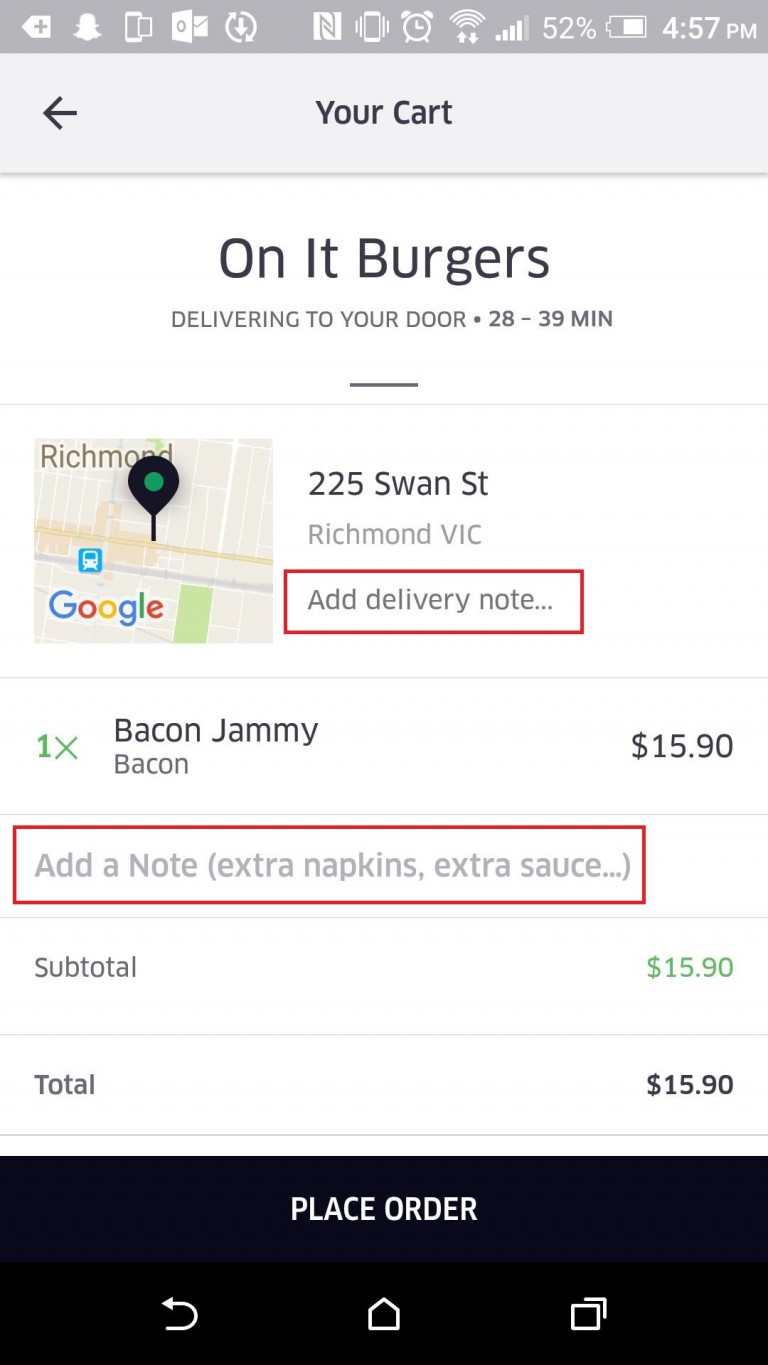**Detailed Caption:**

The image is a screenshot taken from another mobile device, likely an Android phone, as indicated by the familiar icons and layout. The top status bar is a dark gray color, featuring a variety of white icons that include Snapchat, screen sharing, Outlook, a download button, an unknown "N" icon, phone vibrate, an alarm clock, Wi-Fi strength indicator with up and down arrows, a 4 out of 5 signal strength indicator, a battery percentage display at 52%, a battery icon, and the current time displayed as 4:57 PM.

Directly beneath the status bar is a light gray navigation bar with a black left-facing arrow on the far left. Centered along this bar is the label "Your Cart." Below it is a white box containing "On It Burgers" in black text with a subheading, "delivering to your door, 28 to 39 minutes."

Further down, there is a half-screen display showing a Google Maps thumbnail on the left, pinpointed to "Richmond," accompanied by the Google logo. Adjacent to this map thumbnail, the text reads "225 Swan Street, Richmond." Following this is a red-bordered rectangular box with a white background and gray lettering that prompts "Add Delivery Note."

Highlighted in green text below is an order item: "1X Black Letters Bacon Jammie," noted with a price of $15.90 to the right. Another red outline box, this time with white background and light gray lettering, instructs to "Add a Note: extra napkins, extra sauce..." beneath which is denoted the item's subtotal in green at $15.90. Following this is the total amount listed in black at $15.90.

At the bottom of the screen is a prominent black box with white text that reads "Place Order." Finally, the navigation icons for back, home, and recent apps are visible at the bottom of the device's interface.